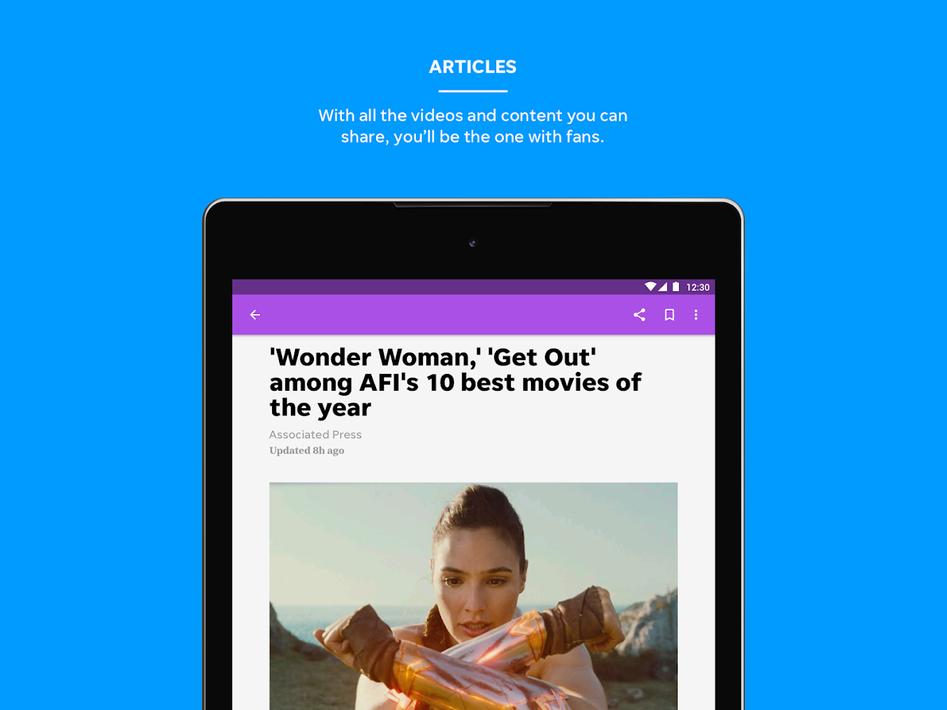The image depicts a vibrant blue background with a solid color scheme. At the top of the image, there is bold text that reads "Articles." Below the text, a tablet or a large smartphone is prominently displayed with black bezels and a centrally positioned front camera at the top edge. The device's screen is actively displaying content.

In the top-right corner of the screen, typical smartphone icons, such as the Wi-Fi signal, battery status, and the time (12:30), are visible. The header of the displayed page is purple, featuring three functional buttons: a share button, a bookmark button, and a menu button, with a back button located at the top left.

The main content of the page shows a white background with black text. The headline reads, "Wonder Woman, Get Out Amongst AFI's 10 Best Movies of the Year," attributed to the Associated Press and marked as updated 8 hours ago.

An image beneath the text features Wonder Woman in her iconic fighting suit, crossing her arms in preparation for a powerful explosion. She is set against a scenic backdrop of a mountain, an ocean, and a sky partially shrouded in light gray clouds. The composition emphasizes a dynamic and engaging visual narrative, perfect for capturing the interest of fans and readers.